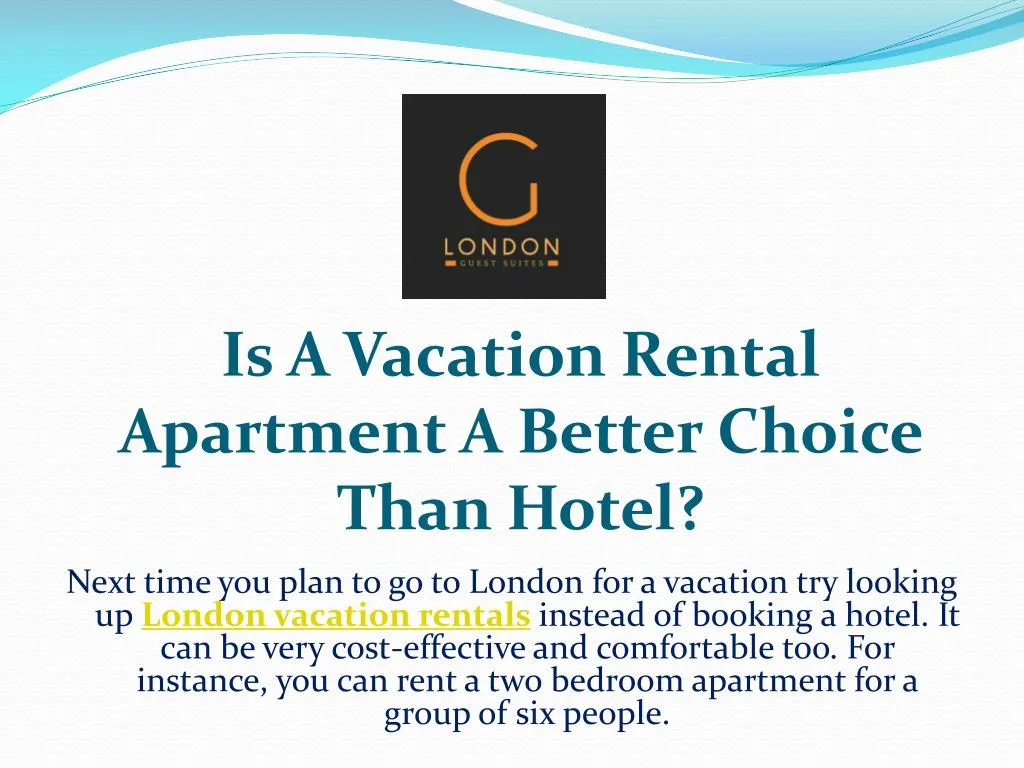The web page features a straightforward design with a visually striking header that mimics the appearance of water, composed of bands of cyan blue and dark blue interspersed with white. At the center of this header is a black square prominently displaying a large, orange letter "G." Below, in a lighter shade of orange, the text reads "London" with an underlined "L" and "N". Beneath that, "Guest Guest Suites" is written in light orange. Further down, in dark teal blue, the tagline "Is a vacation rental apartment a better choice than a hotel?" sparks curiosity.

The body text follows in black, advising travelers, "Next time you plan to go to London for a vacation, try looking up London vacation rentals," with "London vacation rentals" in yellow hyperlink text. The suggestion is that opting for a vacation rental, such as a two-bedroom apartment for a group of six, can be both cost-effective and comfortable. Notably, the capitalization in the phrase "Is a vacation rental apartment a better choice than a hotel?" is inconsistent, with random letters capitalized such as "A," "V," "R," "A," "B," "C," "T," and "H."